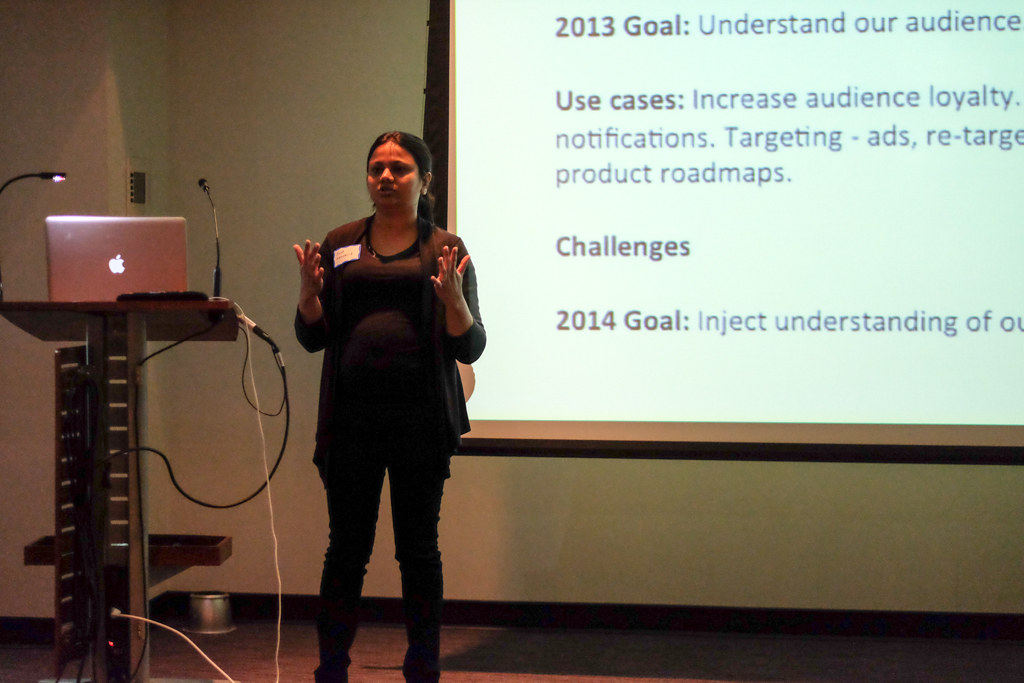In a dimly lit private convention room, a young woman of Indian descent, dressed in an all-black ensemble with a white name tag on her left side, stands in front of a large pull-down projector screen bordered in black. Her hair is neatly tied back in a ponytail, and she is gesturing animatedly, with her fingers spread out in front of her. To her left, a table holds an open Apple Mac laptop, illuminated by a small reading light, and positioned beside a microphone. The projection behind her displays a PowerPoint presentation with the text: "2013 goal: Understand our audience, use cases, increase audience loyalty, notifications, targeting ads, retargeting, product roadmaps, challenges. 2014 goal: Inject understanding," though some words are cut off. The setup, including the content of the presentation, suggests that she is conducting a sales meeting or strategic discussion.